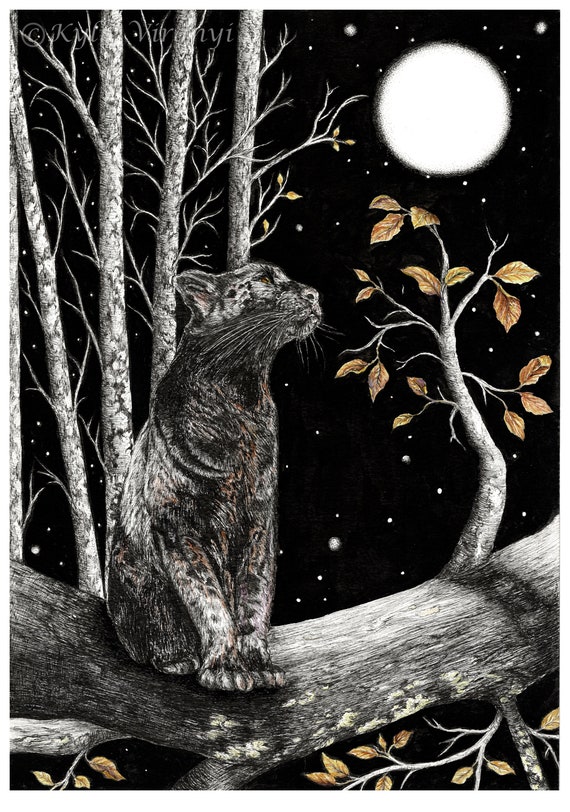The image portrays a serene nighttime scene resembling a wood print, dominated by an intricate interplay of contrasting elements. Central to the image is a black, white, and brown cat, perched near the left of a wide, horizontal gray tree branch that stretches across the foreground. The cat, seated on its haunches with its front paws poised before it and its ears perked up, gazes intently towards the bright white moon in the top right corner of the scene. The moon is set against a completely black sky, dotted with white stars to evoke a starlit night.

The main branch that the cat sits on exhibits multiple smaller offshoots, adorned with bronze-colored leaves, some of which are also sparsely spread beneath the cat. The background features several tall, slender tree trunks, their bark a pale, ashen hue suggestive of aspens, birches, or alders. These trees rise along the left side of the image and are interspersed with wispy branches bearing similar bronze leaves. A subtle hint of moss embellishes parts of the main tree limb, adding texture and depth to the tranquil nocturnal landscape.